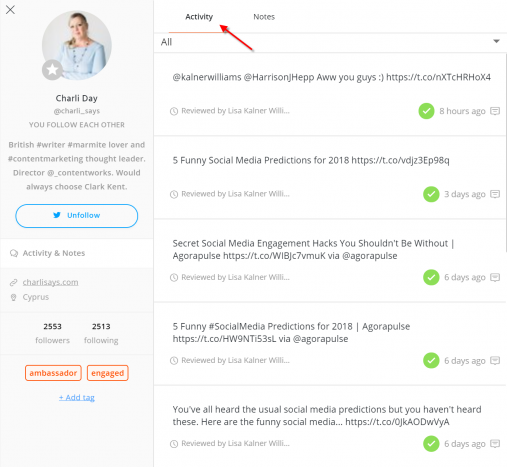Screenshot of a webpage displaying a social media profile of a woman named Charlie Day, with a circular profile picture at the top. Detailed information includes her handle @Charlie_says and shows mutual following status. Charlie Day is described as a British writer, Marmite lover, content marketing thought leader, and director at Content Works. The profile specifies her fictional hero preference as Clark Kent. There is a clickable Twitter unfollow button featuring the Twitter bird icon.

Beneath her profile, the sections "Activity" and "Notes" are visible, with "Activity" being underlined and marked by a red arrow, indicating it is the selected category. The "Notes" section is unselected. Under "Activity," posts include "All you guys :)", "Five funny social media predictions for 2018," and "Secret social media engagement hacks you shouldn't be without," each noted with green check marks. Additionally, options for tagging and buttons to mark as "Ambassador" or "Engaged" are highlighted in orange.